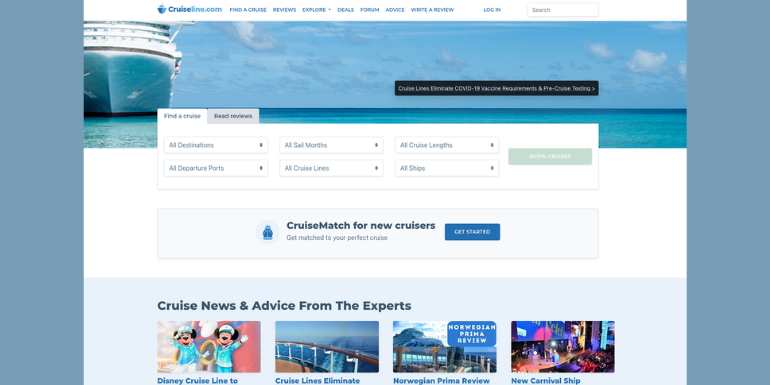This is a screenshot of an advertisement for CruiseLine.com, prominently displayed at the top in blue text. Below the heading, on the far upper left corner, there is an image featuring the bow of a ship. Adjacent to the ship, an expansive blue sky adorned with white clouds stretches to the right, overlaying a rich, deep blue sea beneath.

Part of the sky area is obscured by a black rectangle, rendering its contents unreadable. The lower half of the image transitions to a white background with various selectable categories. Below these categories, the text "Cruise Match for New Cruisers" appears, accompanied by a dark blue rectangular button inscribed with "Get Started" in white text.

Directly below this white area is a section titled "Cruise News and Advice from the Experts," featuring four thumbnail images. The first image shows Minnie Mouse and Mickey Mouse in costume, with the label "Disney Cruise Line" in blue text beneath it. The second thumbnail depicts an onboard view from a ship, overlooking the water, accompanied by the text "Cruise Lines Eliminate." The third thumbnail is labeled "Norwegian Prima Review," showcasing a scenic snapshot with a mountain and water in the background, likely taken from the deck of a boat. The final thumbnail, labeled "New Carnival Ship," is too small to discern specific details from the image.